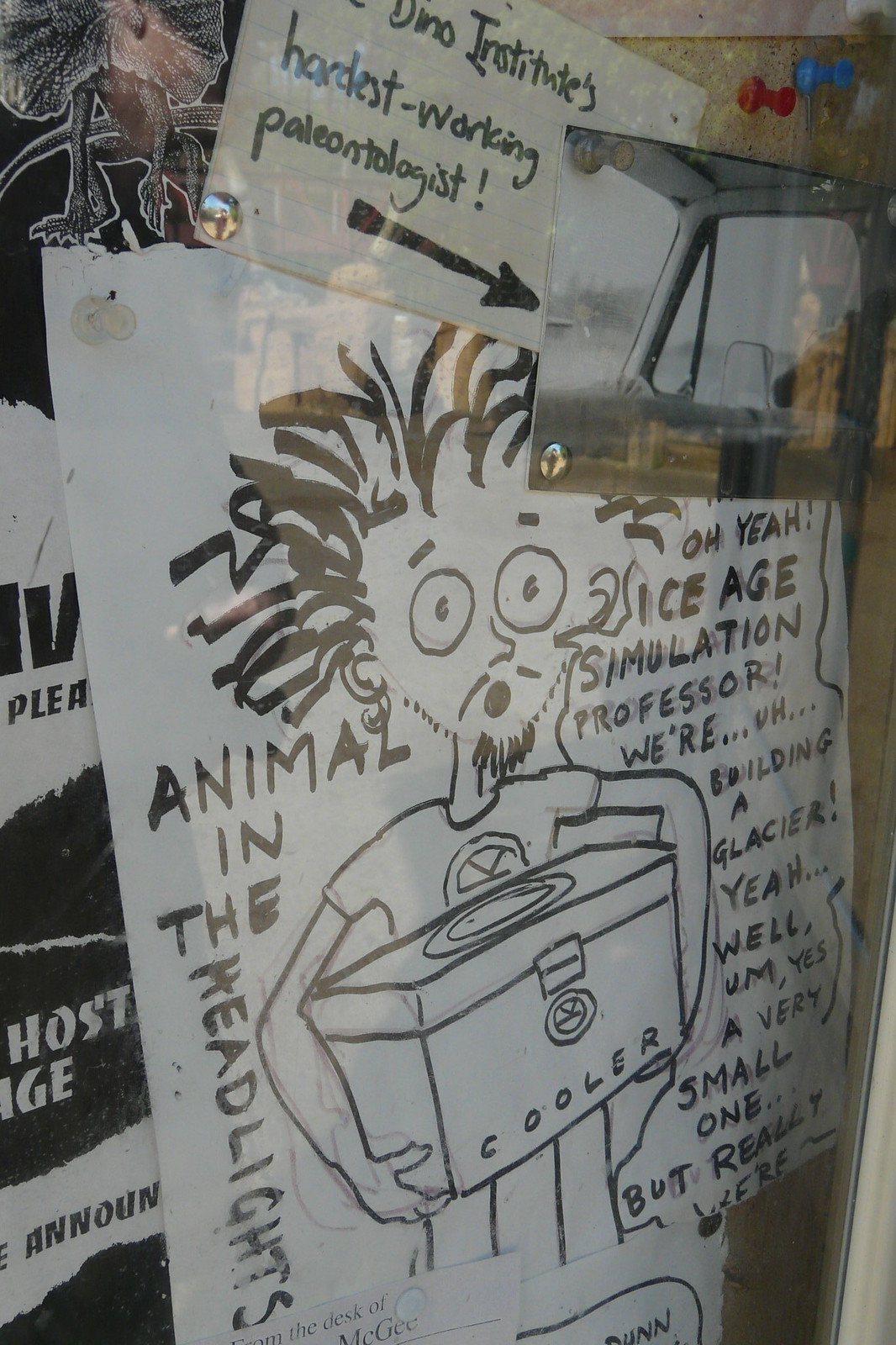The image captures a bulletin board with a clear plastic covering, possibly a corkboard, adorned with various pinned items. Central to the display is a standard letter-sized white sheet of paper featuring a detailed drawing done in marker. The drawing depicts a visibly surprised man with wild, scraggly hair, a goatee, and a mustache. His eyes are wide open, his mouth agape, and he wears a t-shirt while holding a rectangular box labeled "cooler." To the left of him, the phrase "animal in the headlights" is written, and from a speech bubble to his right, it reads, "Oh yeah, ice age simulation professor, we're building a glacier, well yes, a very small one but really we're." The board also includes a postcard-sized white paper with black text written in a Sharpie that says, "Dino Institute's hardest working paleontologist," adjacent to a black arrow pointing right. This arrow directs attention to a black-and-white photograph pinned nearby, depicting the interior of a car, showing a window and side-view mirror. Additionally, in the upper left corner of the board, there is a black-and-white poster partially obscured, seemingly related to dinosaurs, along with a dinosaur sticker enhancing the theme.